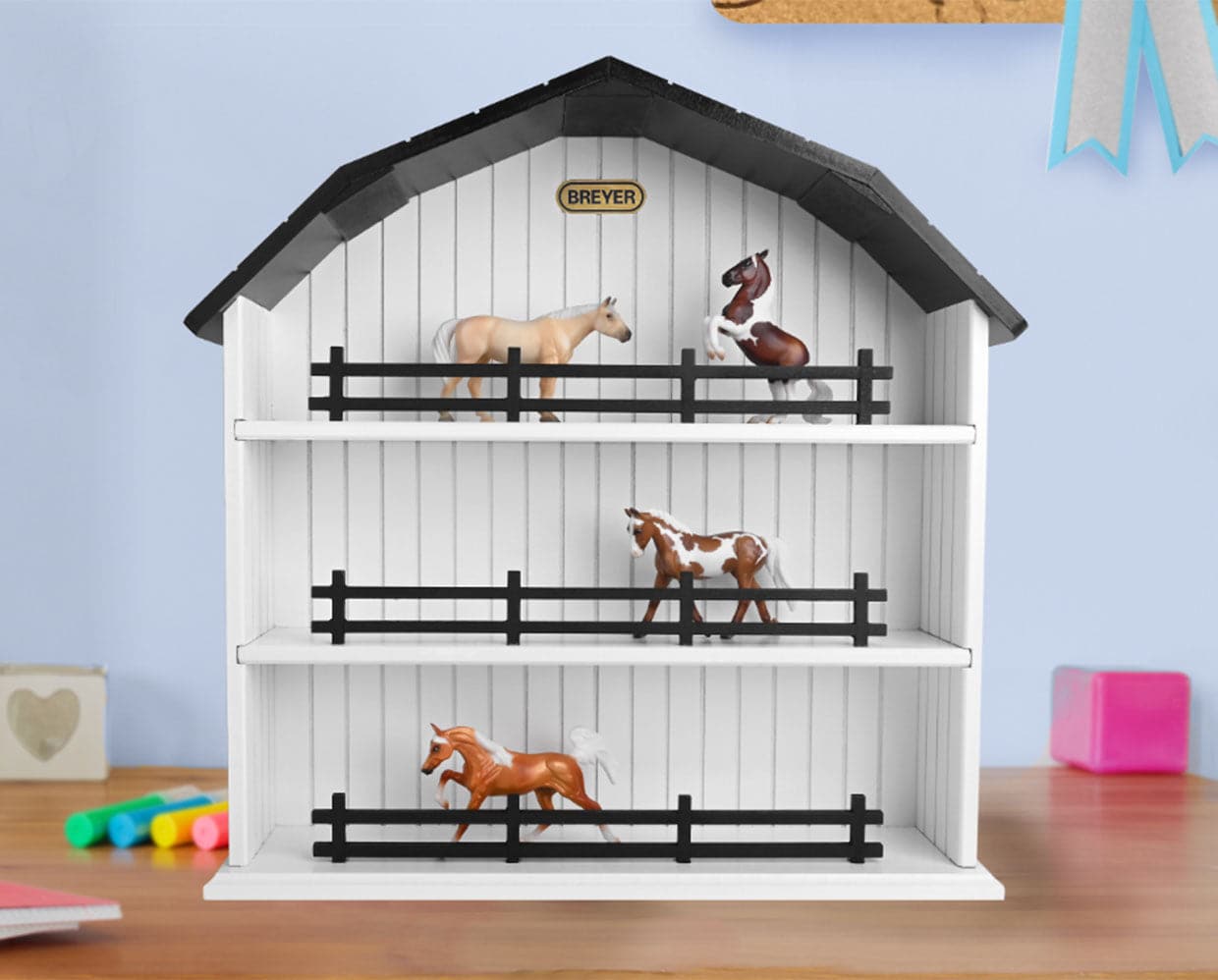This is a detailed photograph of a child's toy barn, designed to resemble a dollhouse but styled as a barn. The barn itself is white with a black roof and sits on a wooden hardwood floor. The structure has three levels, each occupied by toy horses. On the bottom level, there is a chestnut-colored horse with a white mane standing behind a black fence. The middle level houses a paint horse, identifiable by its white coat with brown spots and brown legs, also behind a black fence. On the top level, there are two horses; one is a rearing colt, tan in color, and the other is a standing tan horse. The roof features a sign that reads "Breyer” (B-R-E-Y-E-R), marking the brand of the barn.

The image also includes various other toys and items around the barn. On the left side of the image, there are assorted markers or highlighters scattered on the floor. A pink cube is placed against the pale baby blue wall that serves as the backdrop. Additionally, there is a light gray cube with a heart engraved on it situated on the far left. A ribbon, likely part of a prize or decoration, hangs down from the upper right side of the barn. The colors in the image primarily include black, white, blue, pink, and tan, with the light source originating from the upper left corner.